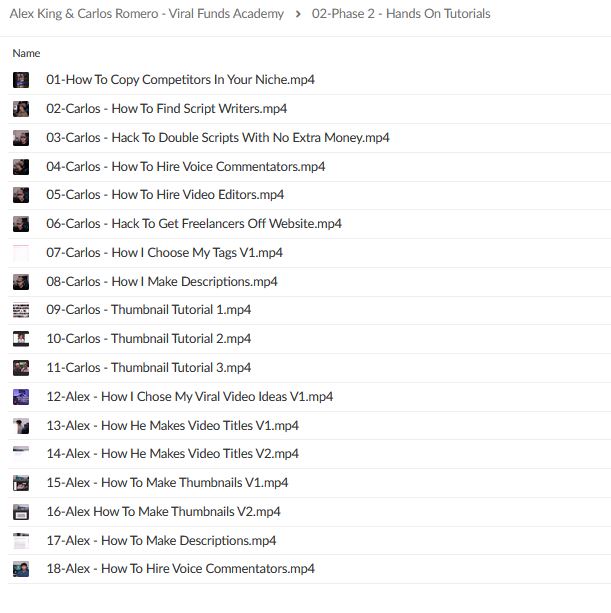The image features Alex King and Carlos Ramiro from Viral Funds Academy prominently at the top. A bold arrow points towards a section labeled "O2 Phase Two Hands-On Tutorials." Below this, there's a listing with a gray line separating the headings from the contents. The list is numbered from 1 to 18, each entry depicting a different tutorial in MP4 format. Each tutorial is associated with a thumbnail image, presumably of screenshots or snapshots of the tutorial contents.

The list includes specific tutorials such as:
1. "How to Copy Competitors in Your Niche" (Carlos)
2. "How to Find Script Writers" (Carlos)
3. "Carlos’ Hack to Double Scripts with No Extra Money"
4. "How to Hire Voice Commentators" (Carlos)
5. "How to Hire Video Editors" (Carlos)
6. "How to Get Freelancers Off Website" (Carlos)

Further down, there is a series of tutorials by Carlos:
- "How I Choose My Tags"
- "How I Make Descriptions"
- "Thumbnail Tutorial"
- Additional Thumbnail Tutorials

Alex King’s tutorials follow:
- "How I Choose My Viral Video Ideas"
- "How I Make Video Titles"
- "How to Make Thumbnails"
- "How to Make Descriptions"
- "How to Hire Voice Commentators"

The layout is clean with white boxes highlighting different sections, providing organized and accessible information on video production topics.